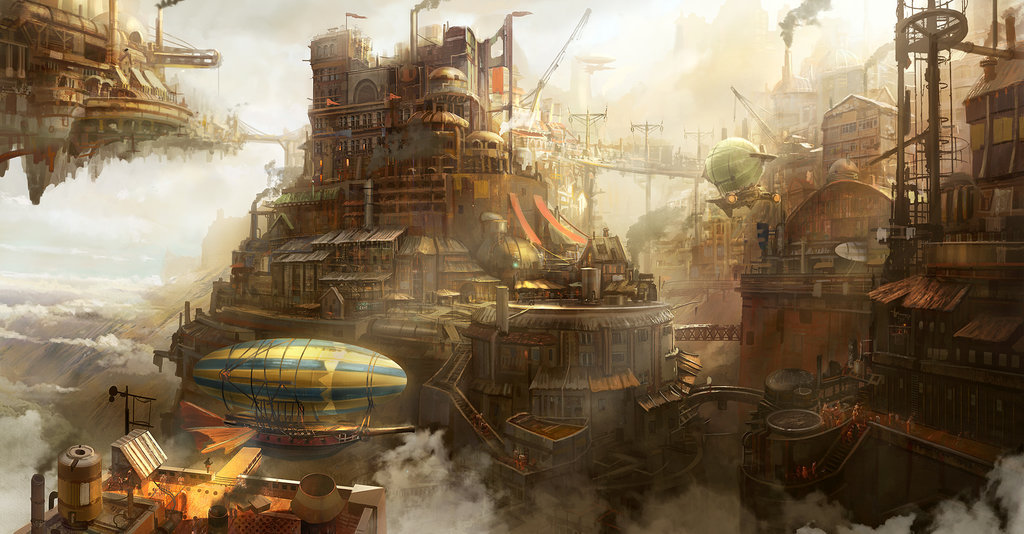This detailed illustration portrays a fantastical and futuristic city suspended within the clouds. Dominated by shades of brown, tan, and grey, the scene features a complex, expansive structure at its center, attached by several bridges to a larger structure extending off the right side of the image. An additional floating segment appears in the upper left corner, connected by another bridge. 

The central structure has a roughly conical shape, encircled by walls and crowned with multiple buildings, chimneys, cranes, smokestacks with billowing smoke, and flags fluttering in the wind, giving it an industrial aesthetic. The atmosphere is hazy, filled with dense clouds, contributing to the misty and dreamlike quality of the illustration.

In the foreground, several airships float gracefully amidst the structures. These blimps, characterized by horizontally striped balloons of yellow and turquoise or blue and yellow, support large, wooden boat-like gondolas. One prominent blimp in the background, adorned with stripes resembling a watermelon, emphasizes the imaginative nature of the scene. The absence of visible people adds to the enigmatic and surreal ambiance of this floating metropolis.